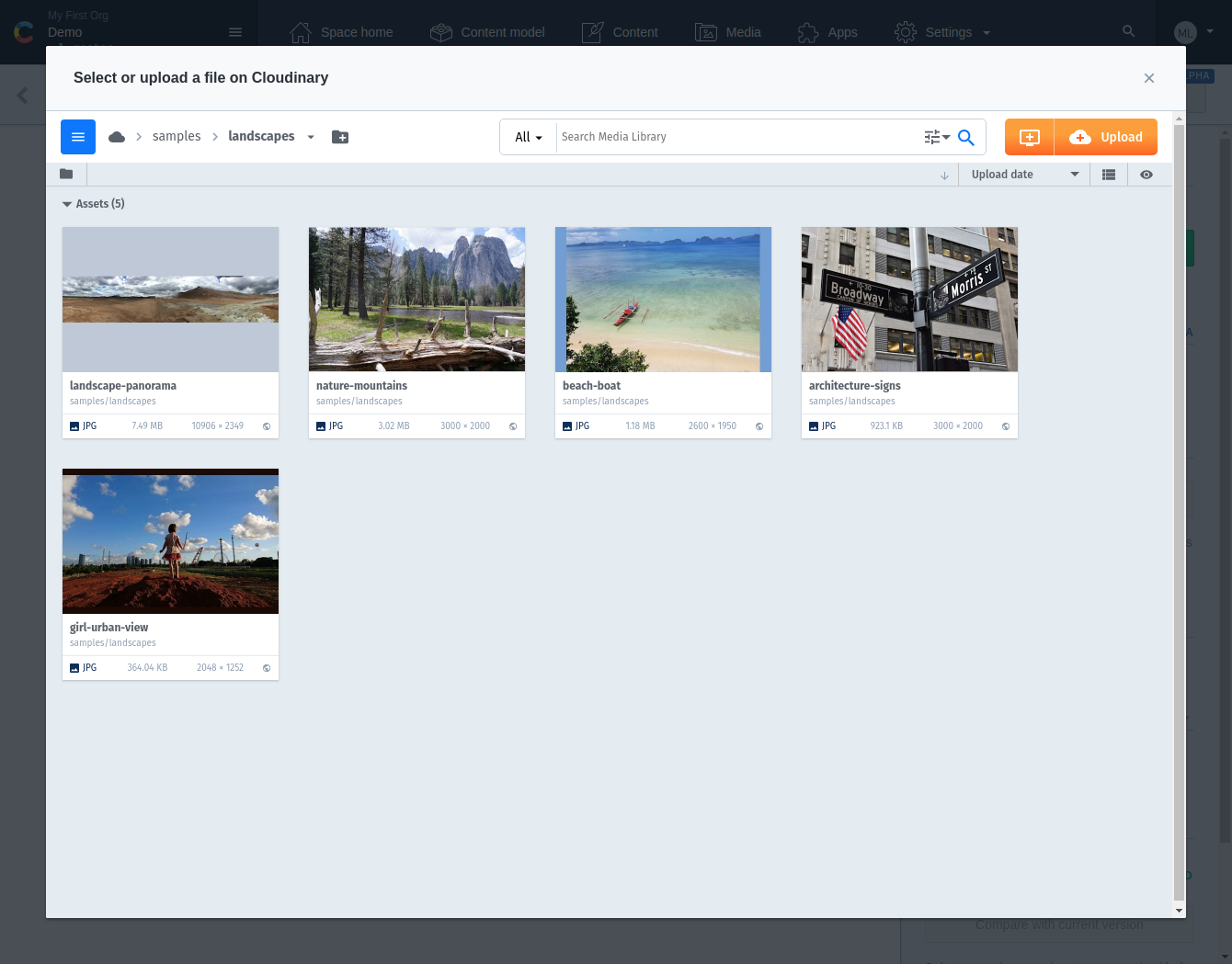This is a screenshot depicting a specific page or pop-up window on a website. The main focus is on the pop-up window, which prominently occupies the center of the image, but the dark grayish backdrop reveals partial details of the underlying web page. At the top-left corner of the background, the name of the website, "Demo," is visible next to a C logo. Above the "Demo" label, it displays "My First Word," while the rest of the menu bar extends to the right.

The menu bar contains several icons: three horizontal lines representing a menu, a house icon for "Space Home," a box icon for "Content Model," a paper and leaf icon for "Content," a picture folder icon for "Media," a puzzle piece icon for "Apps," and a tool icon for settings, accompanied by a drop-down arrow. Additionally, there is a search icon and a circular profile icon with the user's initials to the right.

The pop-up window is labeled "Select or Upload a File on Cloudinary." It features a secondary menu bar with options such as a cloud icon, samples, and landscapes, alongside an upload option represented by a dark folder with a plus sign. Right-aligned on the menu bar is a search bar followed by an orange button labeled "Upload," which shows a cloud and plus sign. Beneath this menu, there are five preview images within the "Assets" tab, displaying various JPEGs of landscapes and nature scenes that have been uploaded.